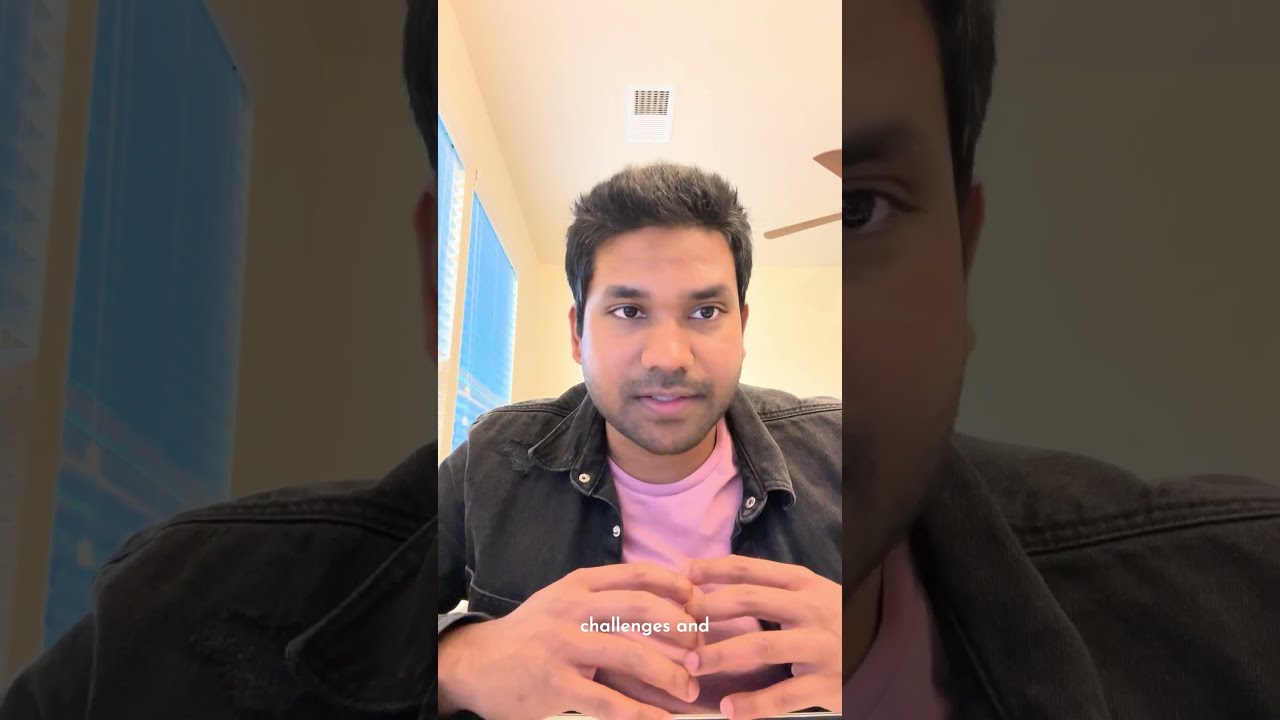The image depicts a handsome, young man of possibly Indian descent with short dark brown hair and light brown, tan skin. He has brown eyes, a small stubbly beard, and a slight mustache. The close-up shot of his face shows him wearing a dark, possibly black, jacket with buttons over a pink shirt. The man is seated inside a room with beige walls and a white ceiling. Above his head, there's an air vent, and the ceiling fan with wooden blades is also visible. He appears to be looking up and to the left, not directly at the camera, suggesting he might be recording himself or watching something off-screen. His fingers are touching together in front of him, and white text reading "and for some reason" is overlaid on the image. Behind his right shoulder, one can see a window with open plastic blinds. The surroundings include multiple perspectives of the man, including a middle panel with his full face and closer views on either side.